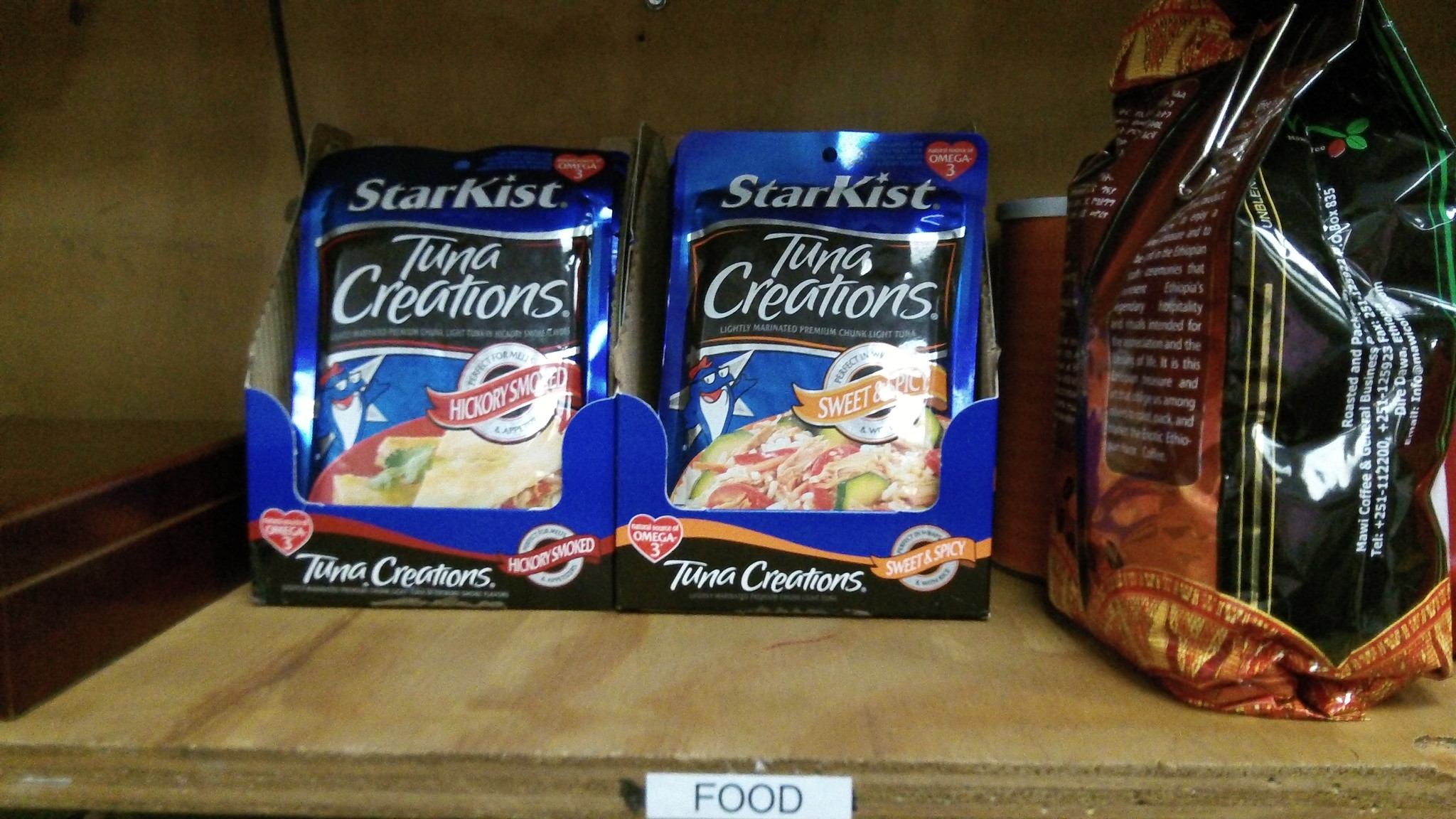This image features a selection of food items arranged on a wooden plywood shelf. Prominently displayed is a small white sign that reads "Food." The focal point of the shelf contains two cardboard display containers for StarKist Tuna Creations, showcasing foil packets in Hickory Smoked and Sweet & Spicy flavors. The blue foil packets bear the recognizable StarKist label, and the accompanying cardboard display boxes are also blue, enhancing brand visibility. Adjacent to the tuna packets is a foil-wrapped bag of Maui Coffee, positioned sideways, making the label with the text "Maui Coffee" visible. The coffee bag adds a touch of exotic flair to the otherwise protein-focused food presentation.